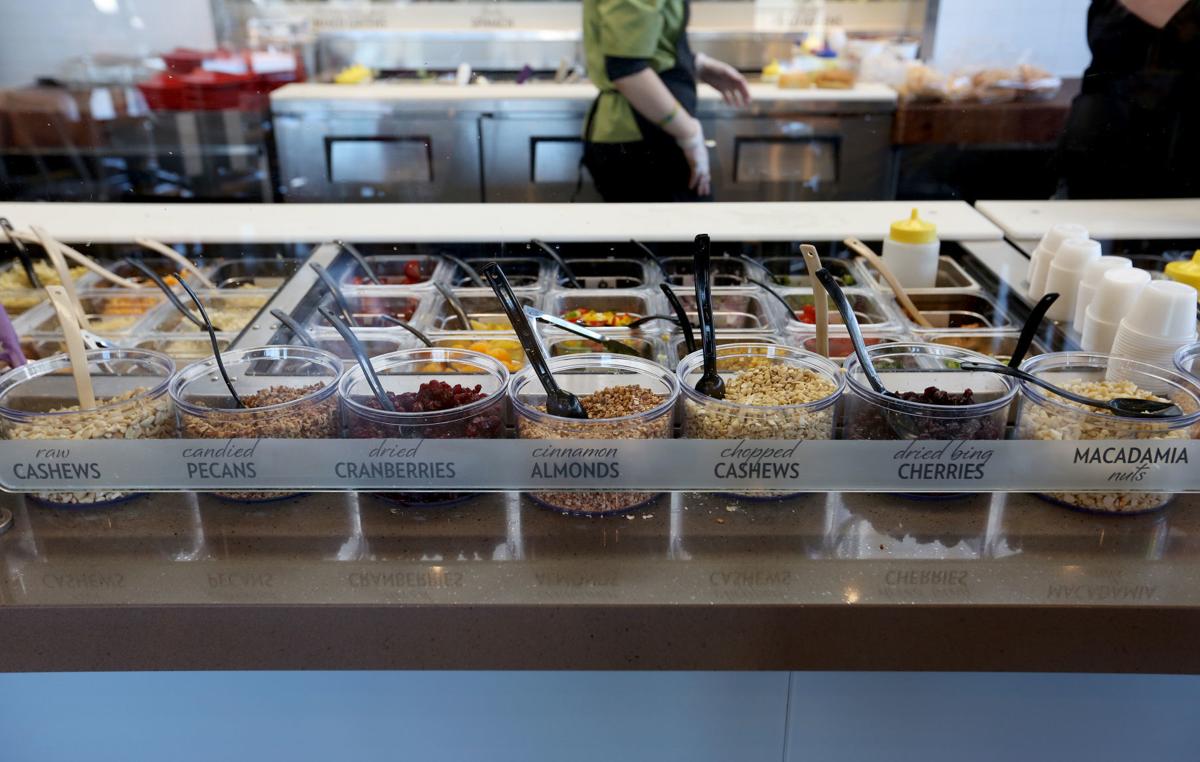A detailed photograph of an interior scene within what appears to be a dessert shop or a toppings bar. The foreground prominently features an array of small, clear plastic cups, each brimming with various chopped and prepared toppings. These include raw cashews, candied pecans, dried cranberries, cinnamon almonds, chopped cashews, dried cherries, and macadamia nuts. Each cup is meticulously labeled with a small, gray rectangular sign displaying the name of the topping.

Behind these dry toppings, an assortment of wet toppings or fruits is visible, carefully arranged in their own containers. This adds a layer of depth and variety to the selection presented.

In the background, the shop's kitchen comes into view. It is equipped with multiple ovens, suggesting a space where lots of baking might occur. A person dressed in a green shirt, black apron, and gloves stands at work, indicating a bustling, functional environment dedicated to preparing delightful treats. The person adds a human element to the scene, anchoring the viewer's attention to the amazing offerings of the shop.